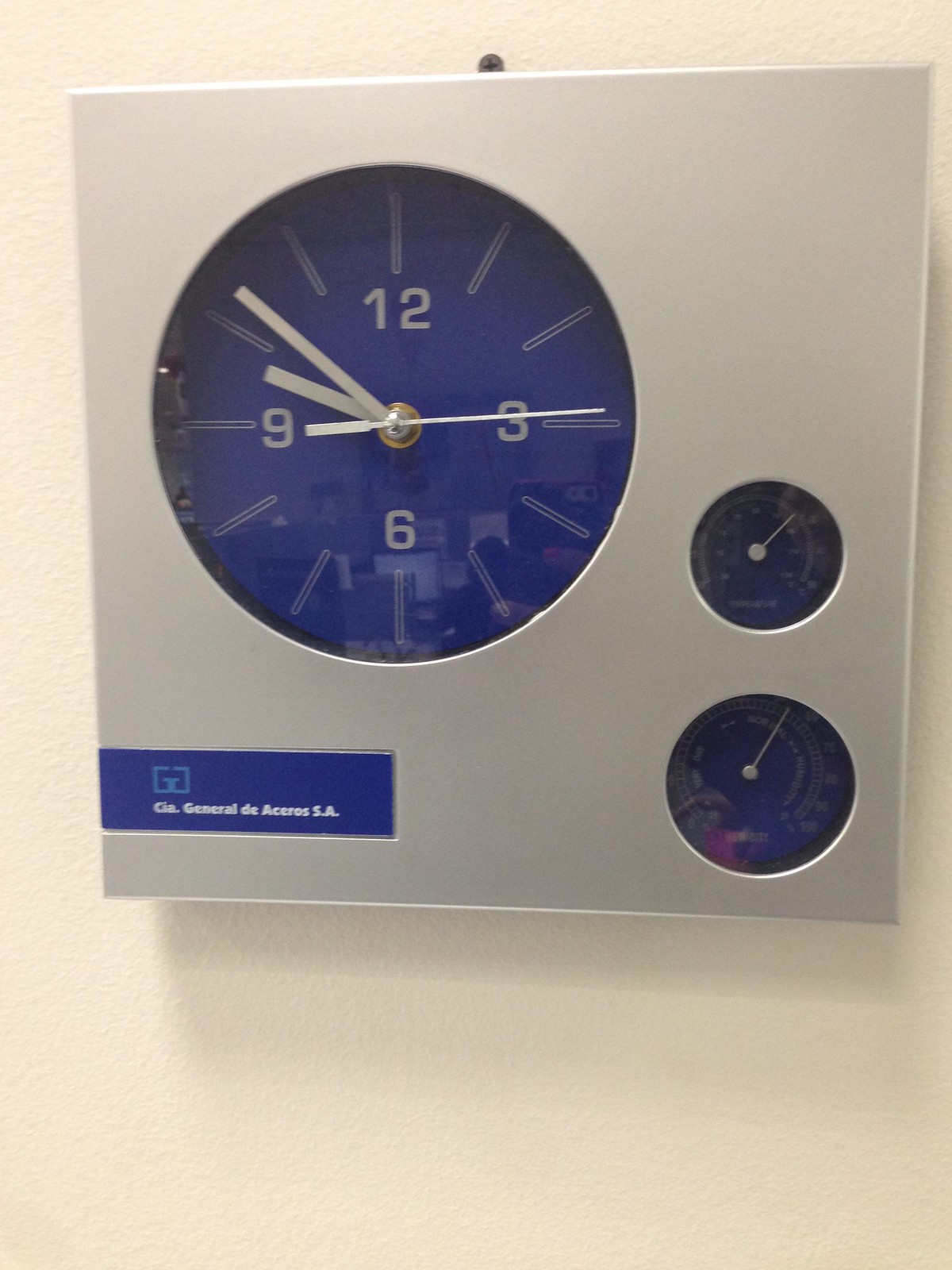This image showcases a sophisticated timepiece set within a sleek square silver case. The primary focus is a blue clock face positioned in the upper left quadrant of the frame. This clock displays the numbers 12, 3, 6, and 9, with simple slashes marking the remaining hours. The clock indicates a time of approximately 9:52, with its hour, minute, and second hands elegantly designed in white. 

Accompanying the clock are two smaller, round instruments located to the right and slightly lower, each about one-eighth the size of the main clock face. The specific purpose of these instruments is unclear due to their diminutive size. 

In the lower left corner of the frame, a small rectangular blue area features printed white text, likely denoting the manufacturer's name. Just above this text is a small turquoise box, adding a subtle touch of color to the overall design.